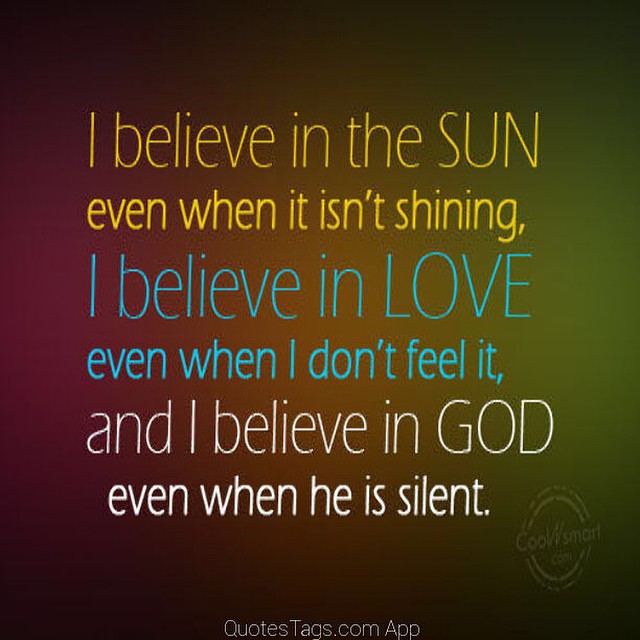This image is a digital illustration from the QuoteTags.com app featuring an inspirational quote. The background has a vignette effect, transitioning from pink on the left to orange, yellow, and green towards the right, with a subtle gradient blending these colors together. The text is split into six lines, alternating between larger and smaller fonts, and uses three colors: yellow, light blue, and white. The quote reads: "I believe in the sun even when it isn't shining. I believe in love even when I don't feel it. And I believe in God even when He is silent." The key phrases "even when it isn't shining" and "even when He is silent" are bolded to stand out. At the bottom center, it's noted as coming from the QuoteTags.com app, and there's a small, somewhat faded circular logo in the bottom right that may belong to CoolSmart.com. The overall effect is a visually engaging and contemplative piece, combining vibrant colors with a message of enduring faith and hope.